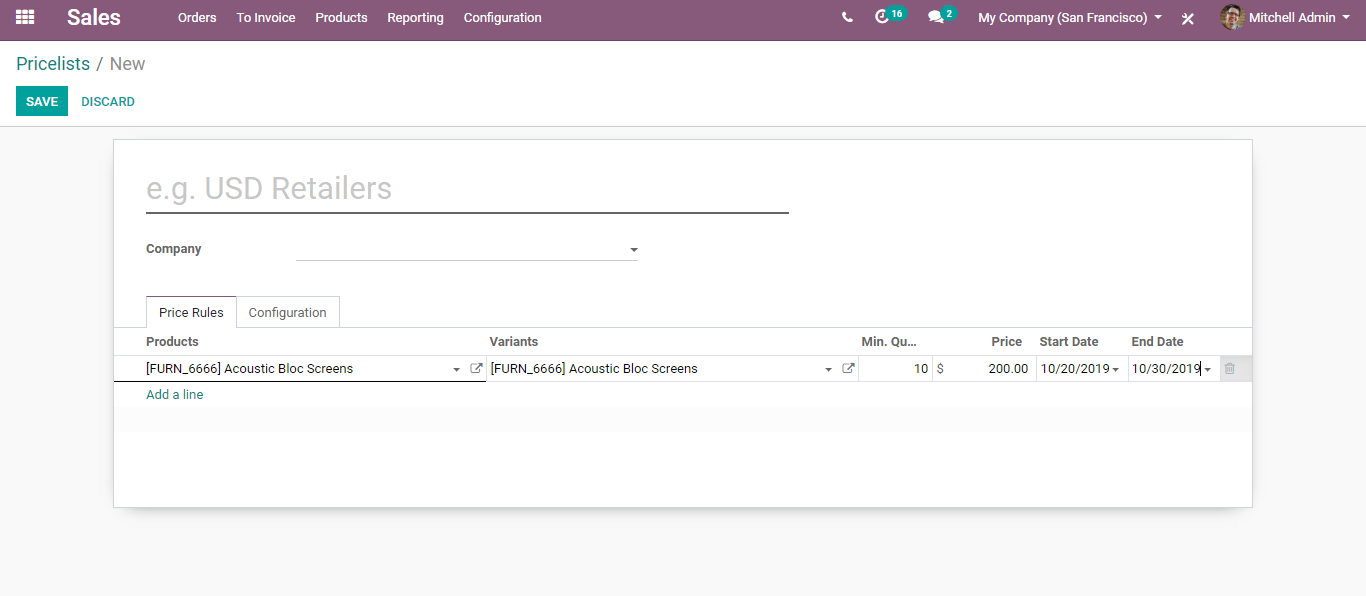The image is a screenshot from a webpage dedicated to sales management. The header is a burgundy rectangle with the word "Sales" prominently displayed. Below the header, there are multiple navigation tabs: "Orders," "To Invoice," "Products," "Reporting," and "Configuration."

At the top of the page, there’s an area indicating "My Company - San Francisco" and the user "Mitchell Admin." Beneath this, there is a section related to price lists, highlighted with the words "Price List" in green, accompanied by green buttons labeled "Save" and "Discard."

The main content area is a large white rectangle showing details like "IEG USD Retailers" and a dropdown menu labeled "Company" for selection. Further down, sections include “Price Rules” and "Configuration."

The "Products" section lists an item "Acoustic Black Screens" priced at $200. The price rule has specified start and end dates: from October 20, 2019, to October 30, 2019.